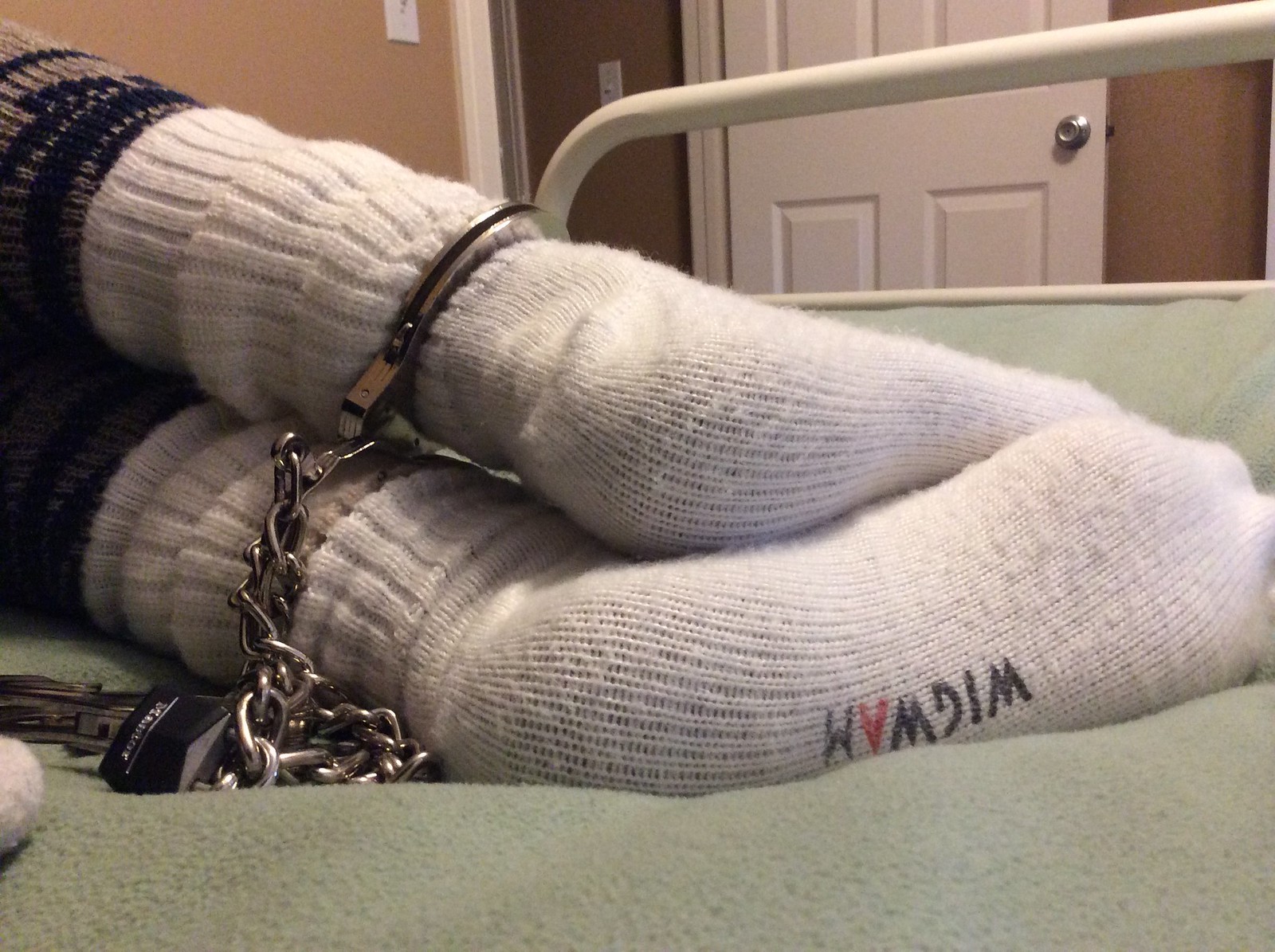This image captures a vivid scene of a person's lower legs and feet lying on what appears to be a bed, possibly a hospital bed. The individual's ankles are secured with silver metal handcuffs connected by chains, with a small black padlock visible on the green bedspread beneath. The feet are clad in thick, ribbed white sports-style socks, typical of winter or athletic wear. Notably, the bottom of one sock features the capitalized word "WIGWAM," with all the letters in black except for a red "A." In the background, a white door with paneled detailing and a silver rounded handle is open, complemented by brown walls that include visible light switches. A hint of a blue and brown textured object is discernible above the socks, enhancing the complexity of the scene.